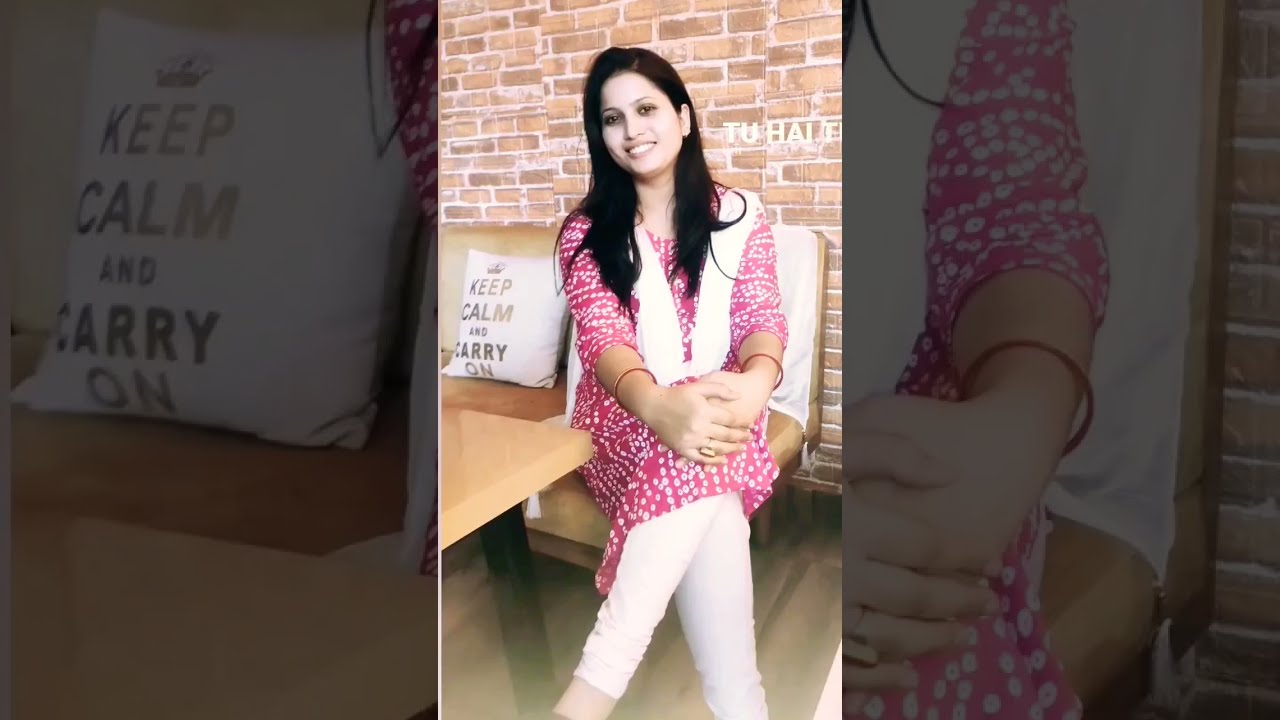The photograph captures a woman with a bright white smile, dark eyes, and long dark hair cascading past her shoulders. She is seated on a fabric chair or couch, with her left leg crossed over her right and her hands clasped over her knee. She is dressed in a long pink dress, adorned with white dots, complemented by white leggings and a white scarf. The woman wears a bracelet on each arm and possibly a hair tie around her wrist. Behind her is a beige pillow with the gold inscription, "Keep Calm and Carry On." The composition of the image is unique, as it is flanked on both sides by enlarged, magnified sections of the central photograph, showing additional details of the pillow and parts of the woman's dress and hands. A brick wall serves as a backdrop, and a table is positioned in front of her to her left.